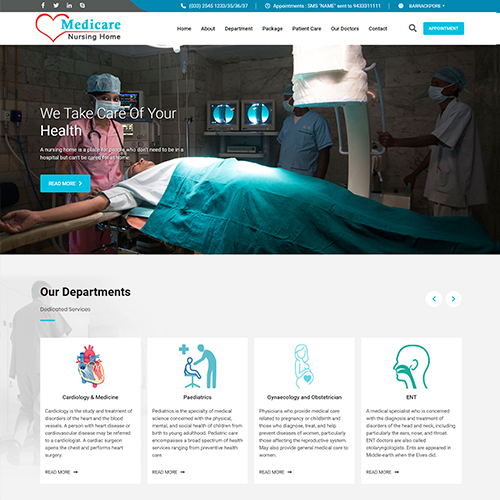The image is a screenshot of a Medicare nursing home website. Dominating the header is the Medicare logo, displayed in blue against a white background. The word "Medicare" is positioned to the right of a red heart outline, which subtly underlines the text by extending the line forming the heart shape. 

To the right of the logo, a navigation menu appears with several options listed. Although the text is small, the menu likely includes tabs labeled "Home," "About," "Departments," "Packages," "Preventive Care," "Our Doctors," and "Contact." Additionally, there is a microscope icon indicating a search function, closely followed by a prominent blue button with white text that reads "Appointment."

Below the header, the main focal point of the image shows a Caucasian man lying on a gurney or medical bed, seemingly being prepared for a procedure. His arms are spread open, and there is a medical professional beside him. The healthcare worker, who appears to be an African American woman, is dressed in pink scrubs, a surgical mask, and a hairnet, and is equipped with a stethoscope around her neck.

Overlaying this scene is white foreground text that reads, "We take care of your health."